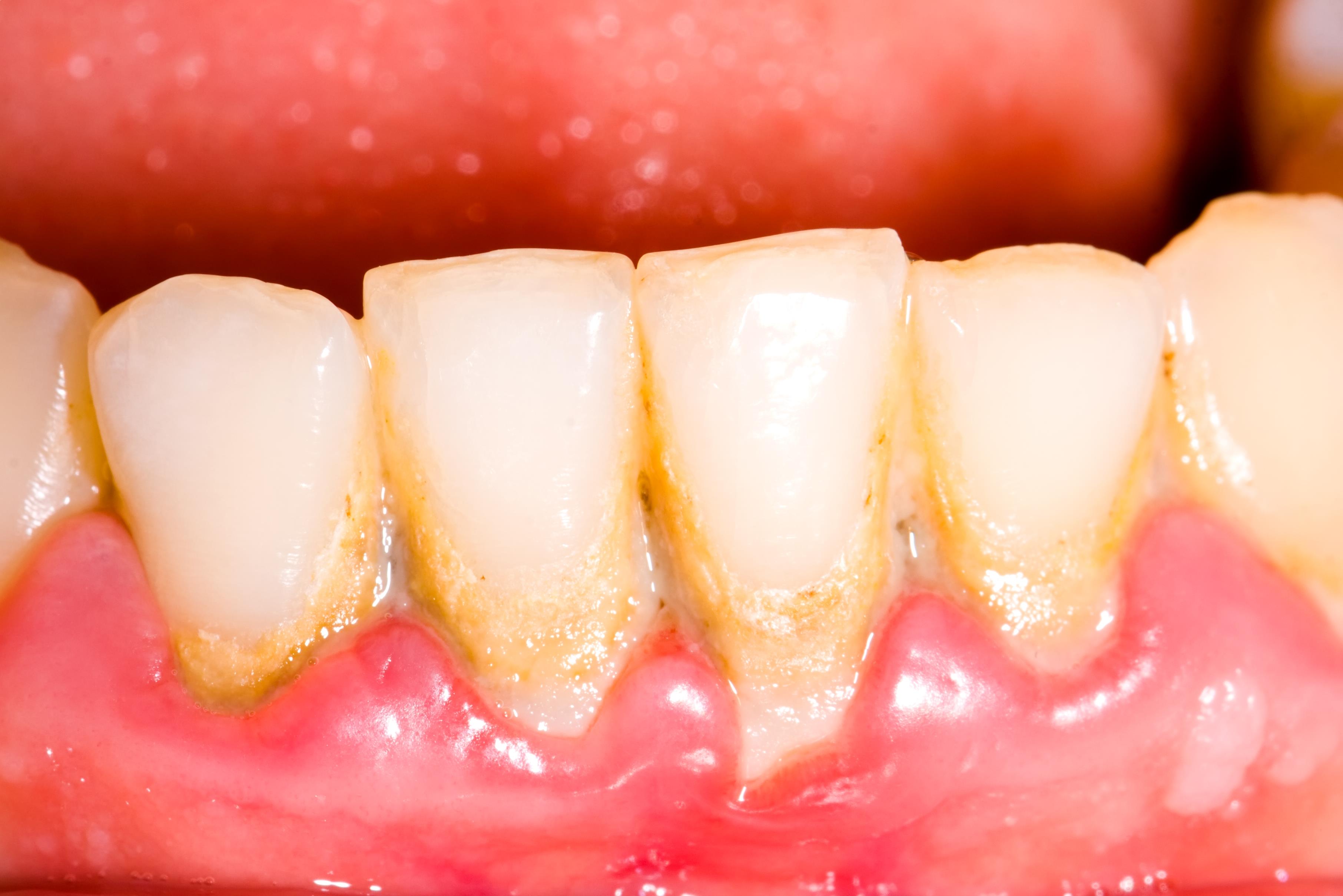The image is an extremely close-up, color photograph showcasing a person’s lower front teeth, specifically focusing on four central teeth. The shot reveals pronounced plaque and tartar buildup around the bases of these teeth, causing them to appear yellowish. The surrounding gums are red and inflamed, suggestive of poor dental hygiene. Additionally, there is a noticeable canker sore on the lower right corner of the individual's lips. The tongue is visible but slightly pulled back, emphasizing the condition of the teeth and gums. The lighting appears to be centered behind the camera, highlighting the severity of the plaque and the need for dental cleaning.